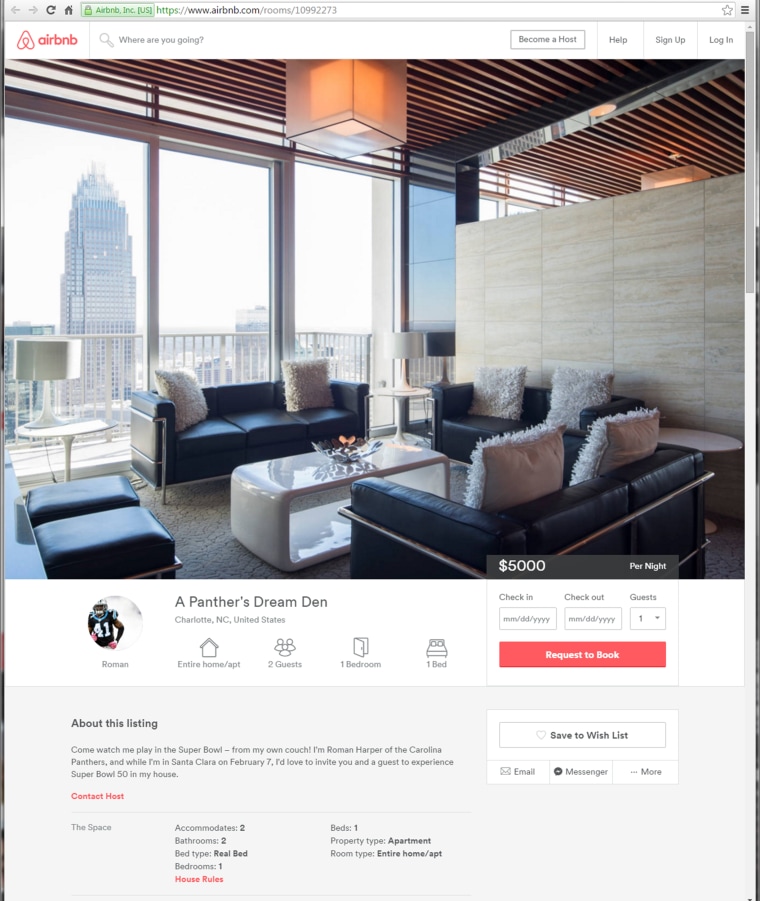The image is a detailed screenshot of an Airbnb listing page. The prominent Airbnb branding is visible at the top with the signature logo—a red symbol accompanied by red "Airbnb" lettering. The URL bar indicates "https://www.airbnb.com/rooms/10992273," and beside it, a secure connection is confirmed by a green rectangle with a green lock and "Airbnb Inc. U.S."

The layout features several elements: a search bar querying "Where are you going?", alongside options to "Become a host," seek "Help," "Sign up," and "Log in." 

Central to the page is a vivid photograph of a luxurious hotel room, adorned with sleek black leather furniture and a modern white coffee table. The room boasts a balcony with a white railing that offers an impressive view of a towering skyscraper. This room, labeled "Panther's Dream Den," is situated in Charlotte, North Carolina, United States.

To the right, within a smaller circular image, there’s a football player donning a black jersey with the number 41. The text beneath the picture identifies him as "Roman." Detailing the accommodation, it states: an "entire home/apartment" for "two guests," featuring "one bedroom" with "one bed." Priced at an extravagant $5,000 per night, the specifics for "check-in" and "check-out" are yet to be filled, and the current guest count is marked as "one." The "Return to request to book" button is conspicuously placed below this section.

Highlighted within a blue background, the listing description reads, "About this listing: Come watch me play in the Super Bowl from my own couch. I'm Roman Harper of the Carolina Panthers, and while I'm in Santa Clara on February 7th, I'd love to invite you and a guest to experience Super Bowl 50 in my house." A red "Contact host" option stands out against the text.

Further details reveal the space accommodates "two guests," with "two bathrooms," a "real bed," and "one bedroom." The "House rules" are marked in red. It additionally confirms the bed count as "one," property type as "apartment," and room type as "entire home/apartment."

On the right, a white rectangle features an option to "save to wish list," yet the hollow heart indicates it is not currently saved. Below this are sharing options for "Email," "Messenger," and "More." Overall, this listing serves as a unique advertisement from Roman Harper of the Carolina Panthers, offering an extraordinary Super Bowl experience at his home.